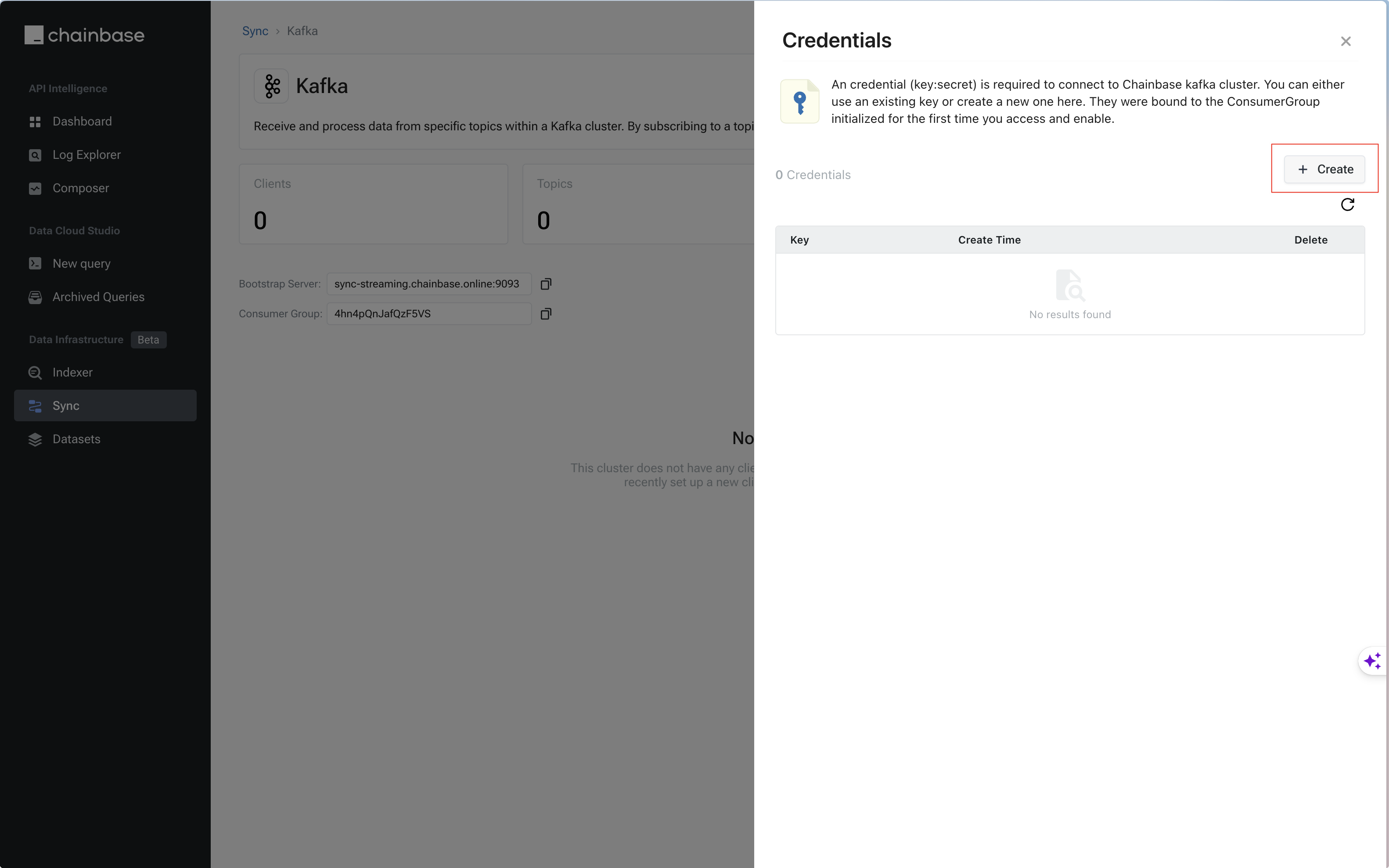The image features a user interface where the left side of the window displays multiple tabs and options against a grayed-out background, likely due to an active pop-up window on the right side. At the top-left corner, it mentions "Chainbase," followed by a message that reads: "Sync Kata: Kata receives and processes data from specific topics within a Kata cluster by subscribing to". Below this, "Client 0" and "Topic 0" are listed.

The left sidebar includes several navigation options: "Dashboard," "Log Explorer," "Composer," "New Query," "Archive Query," and "Indexer." Additionally, there is a section titled "Sync Data Sets."

On the right side of the image, a pop-up window with a white background is open. This window is titled "Credentials" at the top, featuring a close button (an "X") in the top right corner. Below the title, there's an icon of a blue key superimposed on a sheet of paper with a folded upper-right corner. The text below the icon reads: "A credential (key: secret) is required to connect to the Chainbase Kata cluster. You can either use an existing key or create a new one here. They are bound to the consumer group initialized for the first time you access and enable."

This detailed caption offers a clear, comprehensive description of the user interface and its various components as seen in the image.